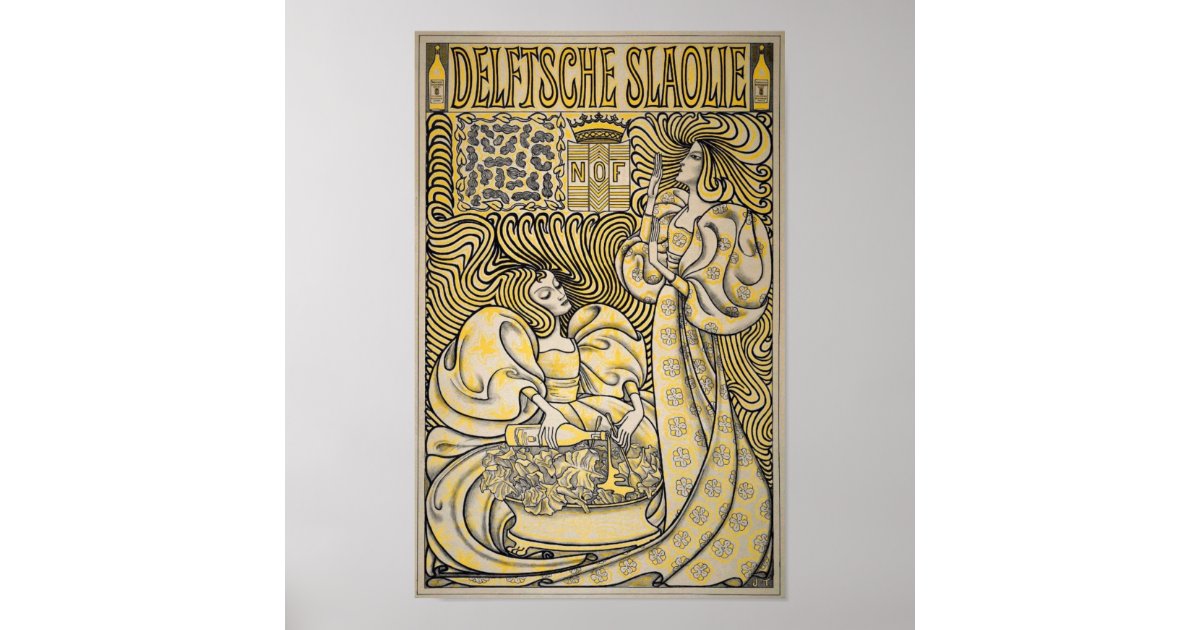The piece is a detailed drawing, primarily rendered in yellows, blacks, and whites, and appears to be either a book cover or a poster. It depicts two regal women, possibly queens, with long, spiraled hair and elaborate, interconnected gowns adorned with floral designs. The woman on the left is seated and pouring yellow liquid from a yellow-colored bottle onto what appears to be a large bowl of plants or a salad. The woman on the right stands elegantly, possibly holding a cigarette, and their flowing hair and gowns create a unique, intricate design that envelops the entire image. Above them, large, creatively stylized yellow text reads "DELPCHE CHALET," flanked by yellow bottles on either side. The background is a grey surface framed in grey, and the top center features a crown, beneath which there's a logo with yellow stripes and designs that reads "N.O.R."